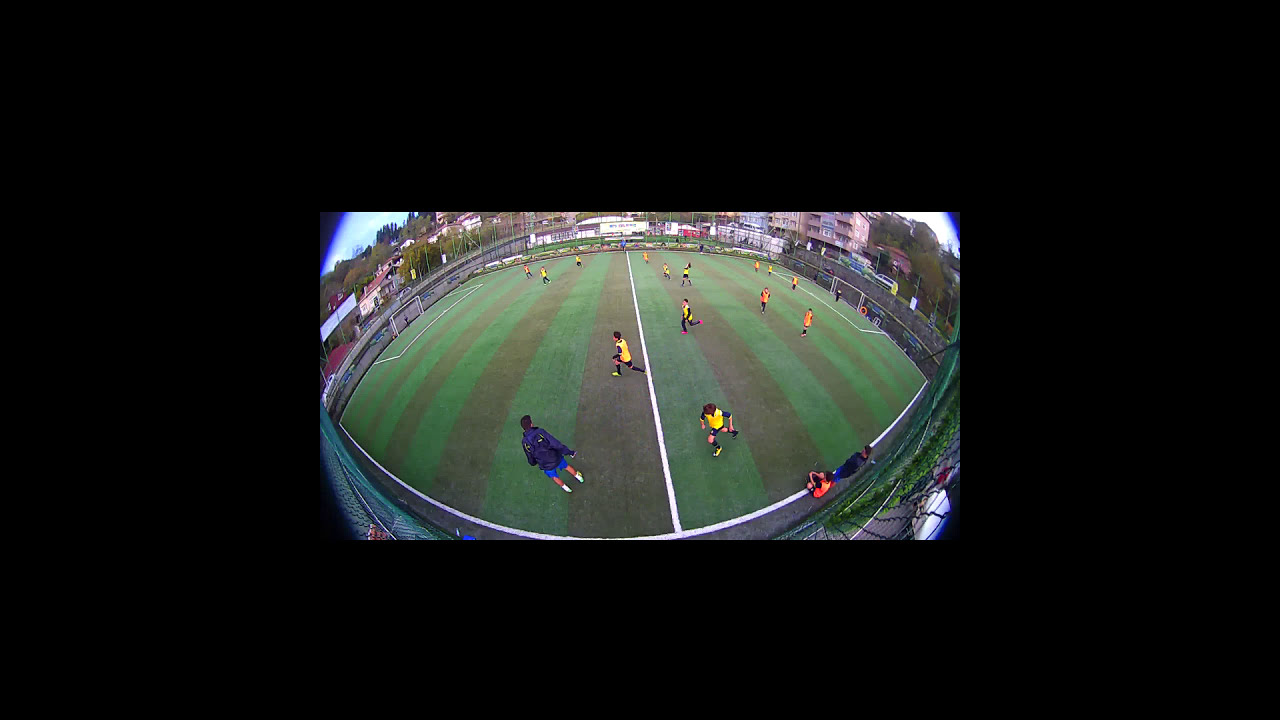The image depicts an aerial view of an active soccer match taking place on a field with alternating light and dark green stripes. The view appears distorted at the edges, likely due to a rounded lens effect, giving a concave impression to the scene. Players in bright yellow jerseys are scattered across the center of the field, actively engaged in the game, while others in orange jerseys are visible on the left side. A figure clad in blue shorts and a black jacket, possibly an umpire or coach, stands prominently in the foreground. Soccer goals are positioned on both the right and left ends of the field. Surrounding the field is some signage and, in the background, a large building can be seen along with distant trees and a glimpse of the sky. The entire image is framed by a thick black border, making the central action appear smaller in contrast. Overall, the setting is outdoors, captured in the middle of the day, with a vibrant mix of colors including black, light blue, brown, red, yellow, green, tan, and gray illustrating the dynamic environment.